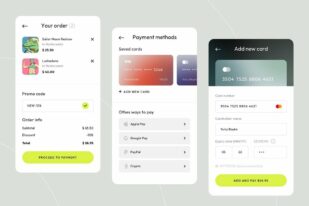The image is a gray rectangle showcasing three staggered screenshots from a cell phone, displayed diagonally from top left to bottom right. The background is predominantly white. 

1. The leftmost screenshot is slightly elevated and shows what appears to be an order summary. The heading "Your Order" is visible at the top, followed by a list of items, possibly video games, each accompanied by colorful images. Money totals are also visible, indicating the cost of each item.

2. The middle screenshot is slightly lower than the first. It displays the heading "Payment Methods" and includes images of credit cards, notably a red card and part of a blue card. The lower section of this screenshot features gray boxes filled with text.

3. The rightmost part of the image includes the upper section of a black cell phone with a gray screen. The screen displays unclear content, potentially a credit card number. Below this, a white overlapping screenshot shows some text boxes and black text, alongside a prominent green-yellow oval button at the bottom, suggesting an interactive element such as a "Submit" or "Continue" button.

The overall composition creates a layered effect, providing detailed visual information about an online purchase and payment process.